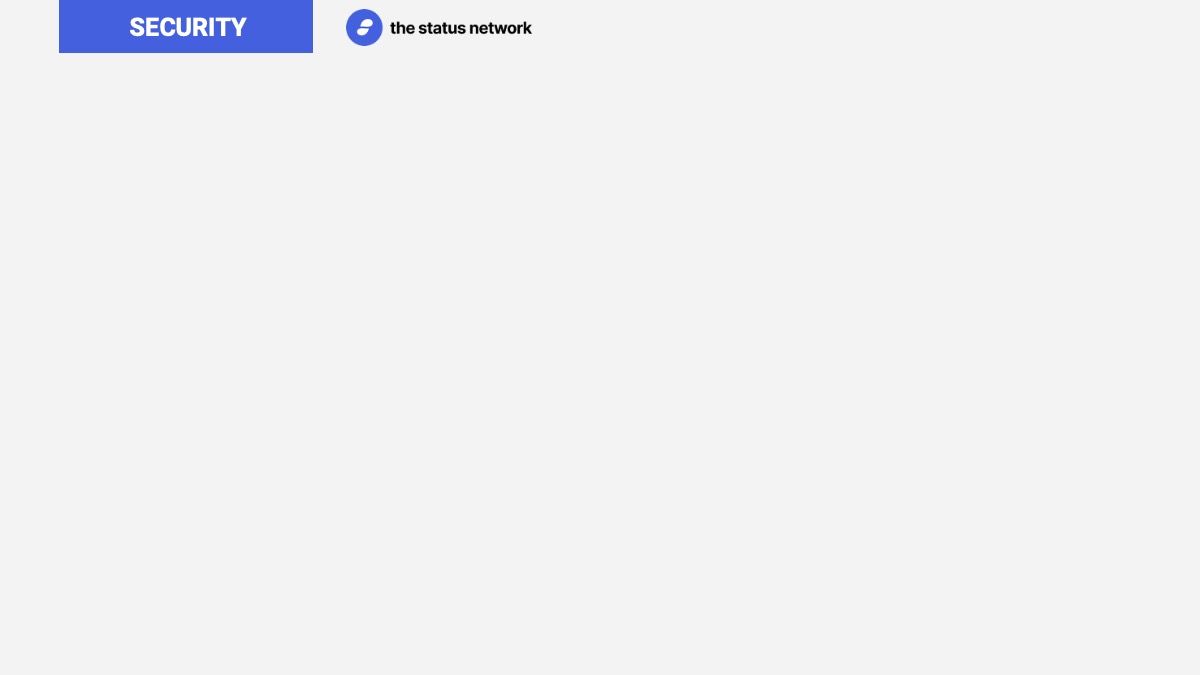The image features a rectangular box with a light gray background, oriented with its longer side running horizontally from left to right. In the top left corner of this rectangle, there is a prominent blue box that stands out against the gray background, containing the word "Security." Moving towards the center of the rectangle, a blue circle is noticeable. Inside this circle is a white icon, although its specific design is not clearly identifiable. Positioned to the right of the blue circle, black text reads "The Status Network." The image is otherwise devoid of additional elements or text.

This visual is meant to be part of a larger narrative, possibly a graphic novel by Christophe J. Belle, aimed at engaging viewers by conveying its thematic essence visually.